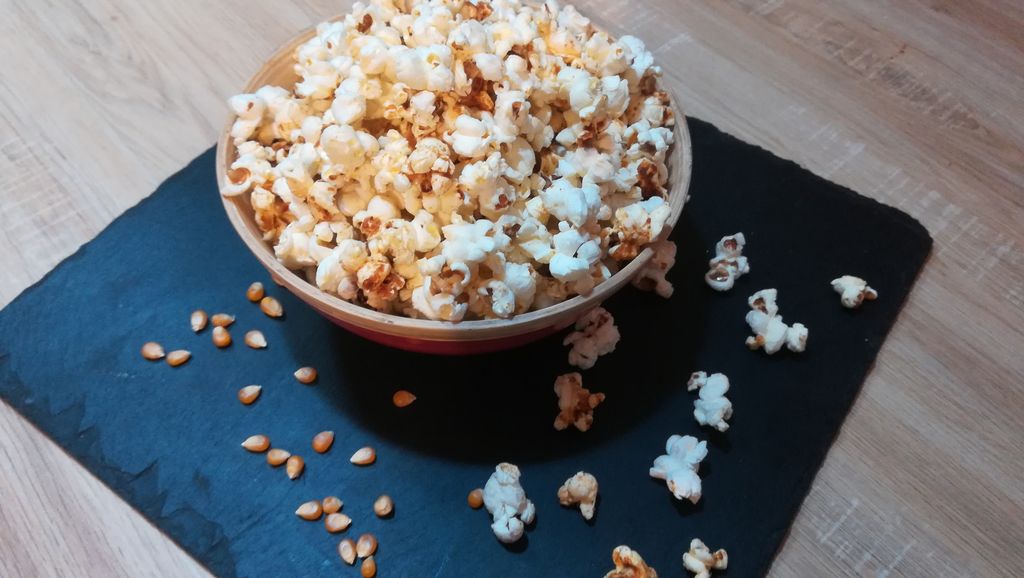The photograph captures a detailed top-down view of a medium brown wooden table, upon which rests a deep blue, frayed-edged slate placemat. Centered on the placemat is a round beige bowl filled to the brim with freshly popped popcorn, some of which has spilled over onto the slate surface. The popcorn is a mix of white and golden kernels, and there's a notable quantity of unpopped kernels scattered particularly towards the bottom left-hand side of the placemat. The bowl, which features a pink hue with a white rim and a hint of gold, has its diameter measuring approximately three-quarters of a foot. The overall scene suggests a casual, slightly messy serving of popcorn ready to be enjoyed.